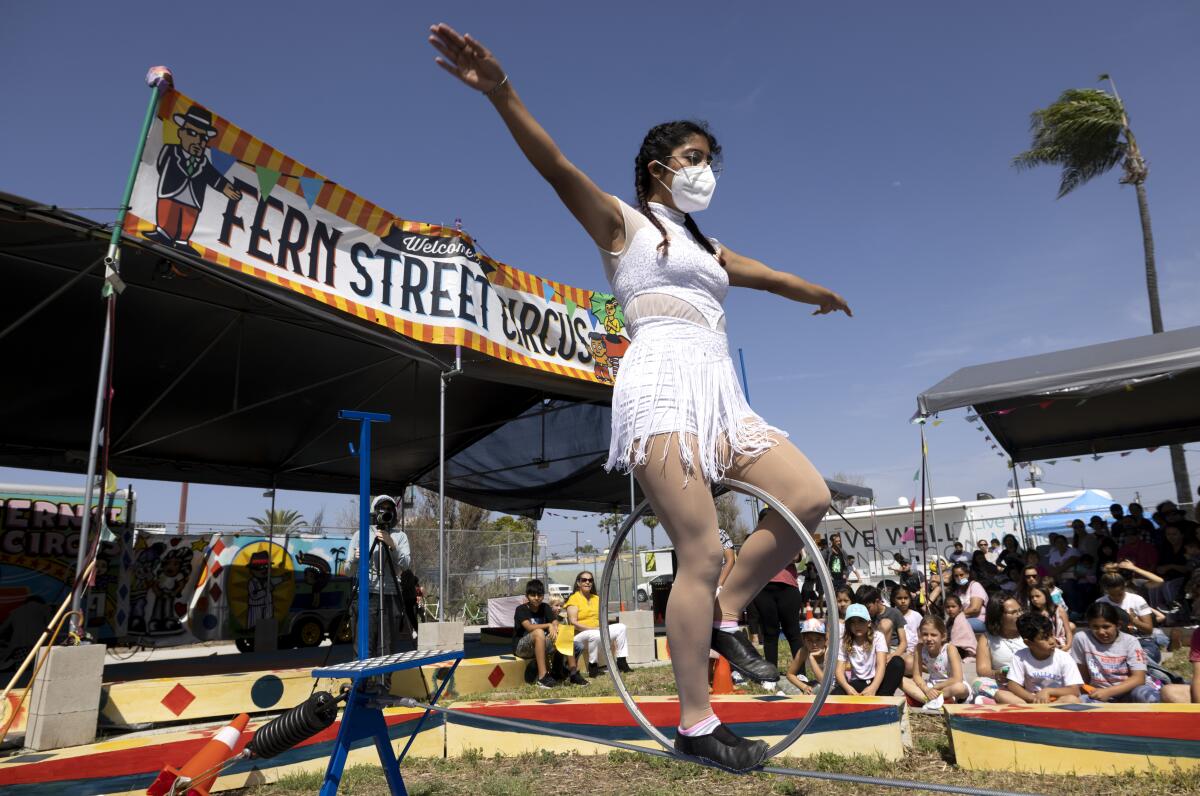In the vibrant outdoor setting of the **Fern Street Circus**, a talented female performer with tan skin is captured mid-performance on a silvery unicycle, which is delicately balanced on a tightrope. She exudes grace and confidence, her arms raised in the air, donning a white fringed outfit consisting of shorts and a string top, paired with black shoes. Her face is partially obscured by a COVID-era mask. Behind her, a sign with the black text "Fern Street Circus" stands out against a white background adorned with vertical orange and yellow lines. The backdrop features lush green palm trees under a clear blue sky. Spectators are seated beneath tents and small bleachers, engrossed in the performance, completing the lively circus atmosphere.